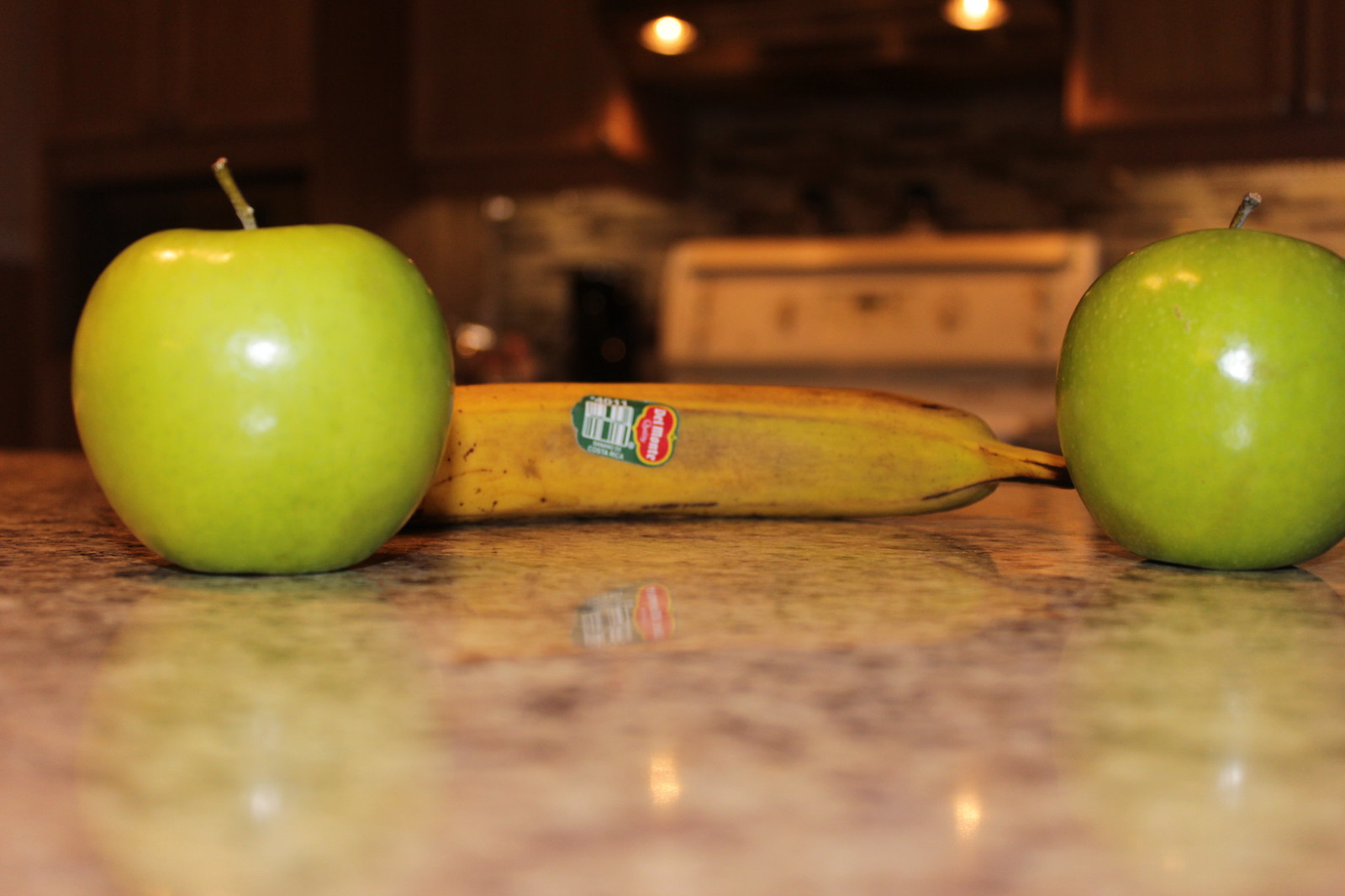At counter height, the camera captures an intimate and detailed view of a kitchen counter scene. The very bottom edge of the image is blurred, creating a soft focus effect that contrasts with the crisp detail of the focal objects: two glossy green apples, each adorned with a stem. Positioned between the apples is a well-ripened banana, its yellow peel speckled with multiple brown marks suggesting it's slightly overripe. The banana bears a distinctive Del Monte label. This label features a red background bordered with yellow and green, with the name "Del Monte" prominently displayed in white font and a UPC section in white at the bottom.

In the background, though blurred, a kitchen setting is discernible. A white stovetop and oven occupy the space, framed by kitchen cabinets overhead. A tiled backsplash provides additional texture, with a mosaic of brown and gray hues adding a touch of elegance.

The countertop below the fruit, likely crafted from marble or quartz, shows their reflections clearly, including the Del Monte sticker, further emphasizing the polished surface. This reflective detail adds depth to the image, enhancing the realism of the scene.